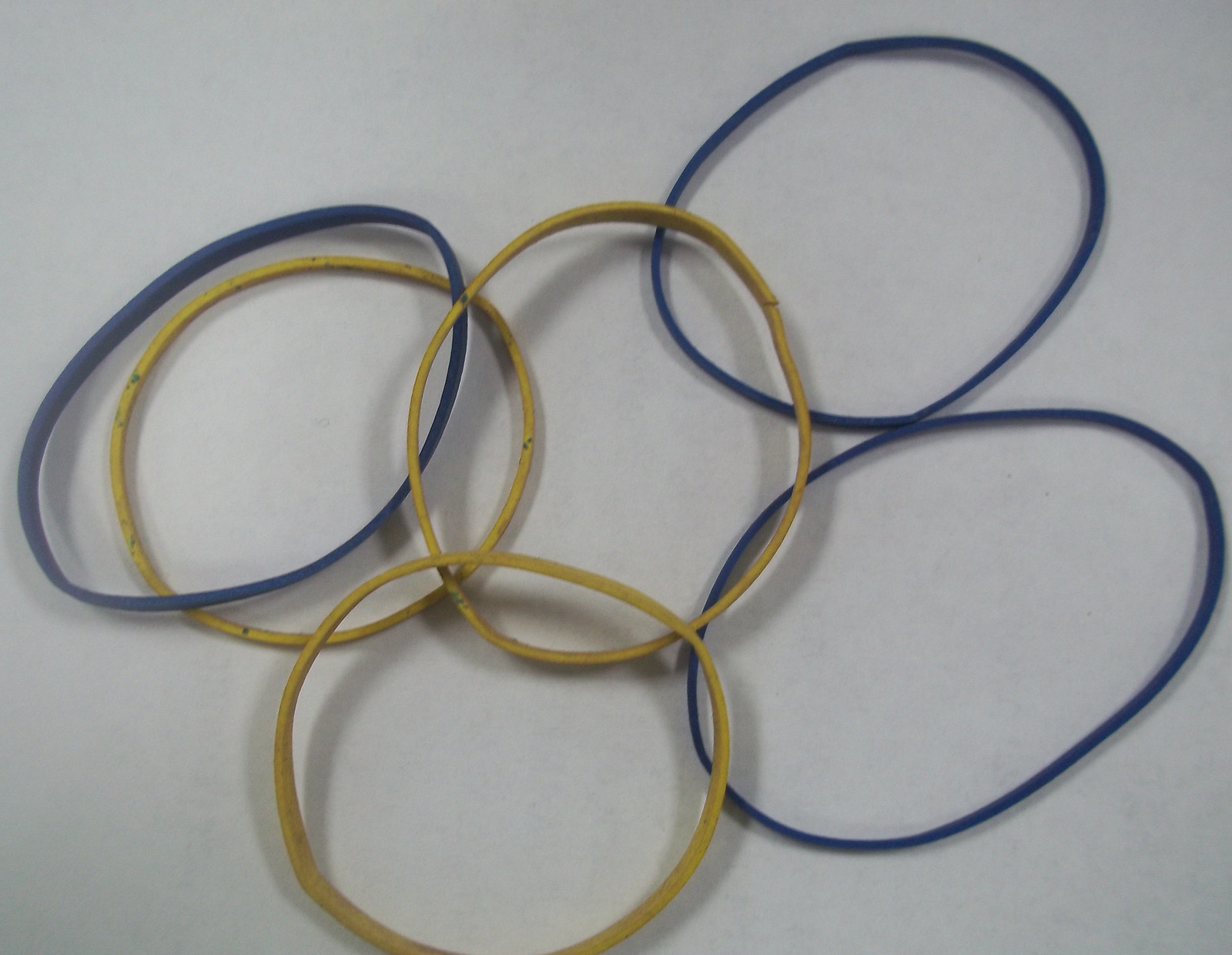This is a detailed photograph featuring six rubber bands, three blue and three yellow-brown, arranged on a stark white background. The yellow-brown rubber bands are centrally positioned, with one at the top overlapping another at the bottom left, forming a triangular shape. The blue rubber bands are more scattered; one is diagonally placed in the left center, another is slightly rounded in the upper right underneath the yellow-brown bands, and the third is positioned diagonally in the middle to lower right, also under the yellow-brown ones. Shadows from the rubber bands indicate the presence of light, adding depth to the composition. The rubber bands measure approximately three to four inches in diameter.